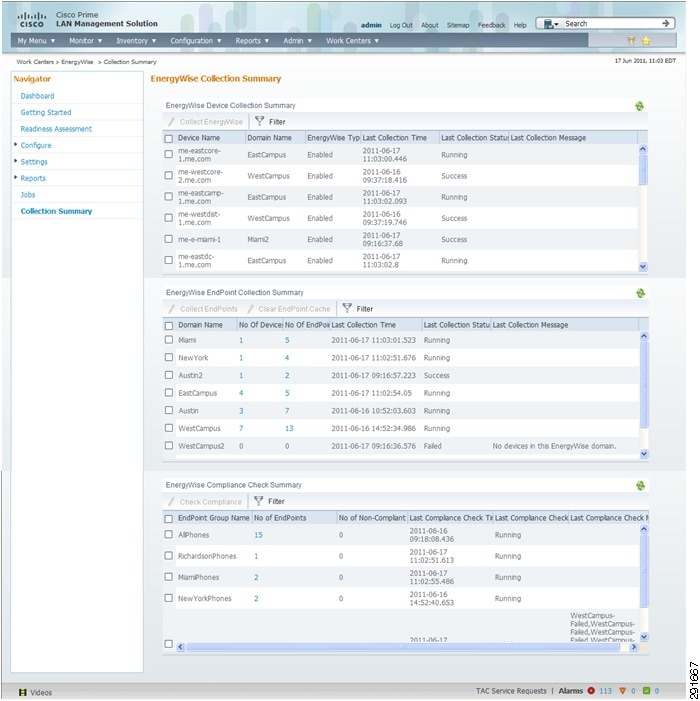The image depicts a comprehensive dashboard titled "Cisco Prime LAN Management Solution." At the top left, the header bears the title in bold lettering. To the right, user options are available including "Admin," "Log Out," "About," "Sitemap," "Feedback," and "Help," accompanied by a search bar for easy navigation. Below the main header, a navigation menu offers various sections: "My Menu," "Monitor," "Inventory," "Configuration," "Reports," "Admin," and "Work Centers."

Further down, a secondary menu presents additional categories: "Navigator," "Dashboard," "Getting Started," "Readiness Assessment," "Configure," "Settings," "Reports," "Jobs," and "Collection Summary." Adjacent to these categories, there are three distinct information sections.

The first section, titled "Energy-Wise Device Collection Summary," offers a detailed collection of device data. Below this is the "Energy-Wise Endpoint Collection Summary," listing specific endpoints such as "Miami," "New York," and "Austin 2." The final section, "Energy-Wise Compliance Check Summary," provides further compliance-related details. Each segment is structured to offer a summary, enhancing the user’s ability to manage and assess various aspects of network performance and energy efficiency effectively.